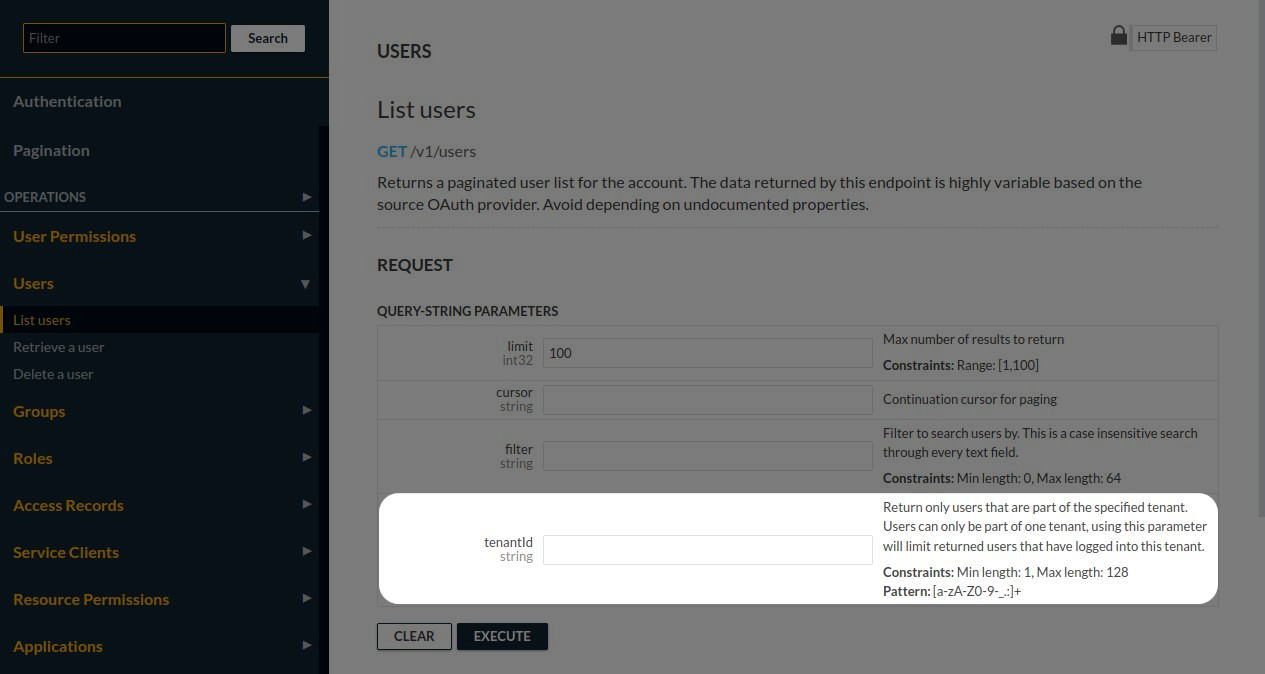This image depicts a website interface, slightly blurred but still discernible. The left side of the interface features a vertical black bar that runs down the length of the page. At the top of this bar is a search function. Below the search bar, the sidebar lists various sections in alternating orange and white text, including "Authentication," "Pagination," "Operations," "User Permissions," and "Users."

The main content area of the website prominently features the word "Users" at the top. In the upper right corner, there's a lock icon alongside the text "HTTP Bearer." Directly below this, the heading "List Users" appears, accompanied by an HTTP GET request formatted as "GET /users." A descriptive note informs that the endpoint returns a paginated user list for the account and advises against depending on undocumented properties due to the variability based on the source authentication provider.

Beneath this, the section titled "Requests" details "Query String Parameters," displaying several input boxes. Most of these boxes are highlighted in gold, except the final one. The last box includes text specifying that only users part of a specified tenant should be returned, indicating that users can belong to a single tenant only. This implies that using this parameter will limit the returned users to those associated with the specified account.

At the bottom of the section are two buttons labeled "Clear" and "Execute," enclosed within a prominent white outlined box, possibly indicating their interactive nature or prominence in the interface functionality.